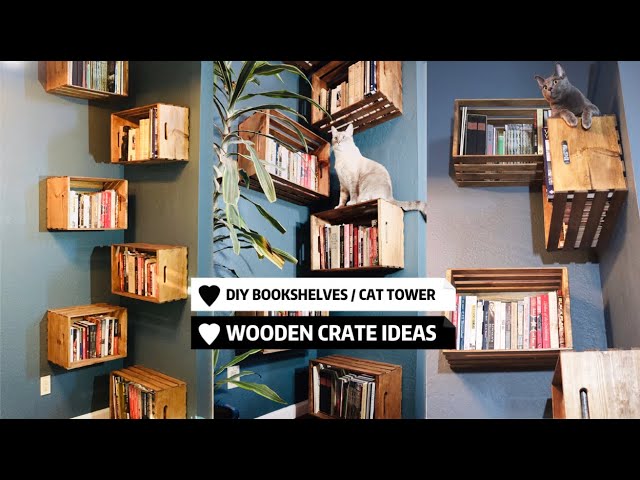The image prominently features two text boxes in the center: a white rectangle with black text that reads "DIY Bookshelves / Cat Tower" featuring a black heart, and a black rectangle with white text that reads "Wooden Crate Ideas" with a white heart. Both text boxes have their upper right corners folded down like pieces of paper. The background showcases a creative setup where wooden crates have been affixed to a wall, serving dual purposes as both bookshelves and a climbing cat tower. The wall itself transitions from a green zigzag pattern on the left to a gray tone on the right. The crates are arranged in a stair-like pattern, allowing cats to hop from one to another. The central crate holds a gray cat with a white neck, and another gray cat can be seen on an upper-right crate. Additional details include a green plant positioned slightly left of center amidst the crates, multiple crates filled with books, and various wall sections that reveal the room's decor.